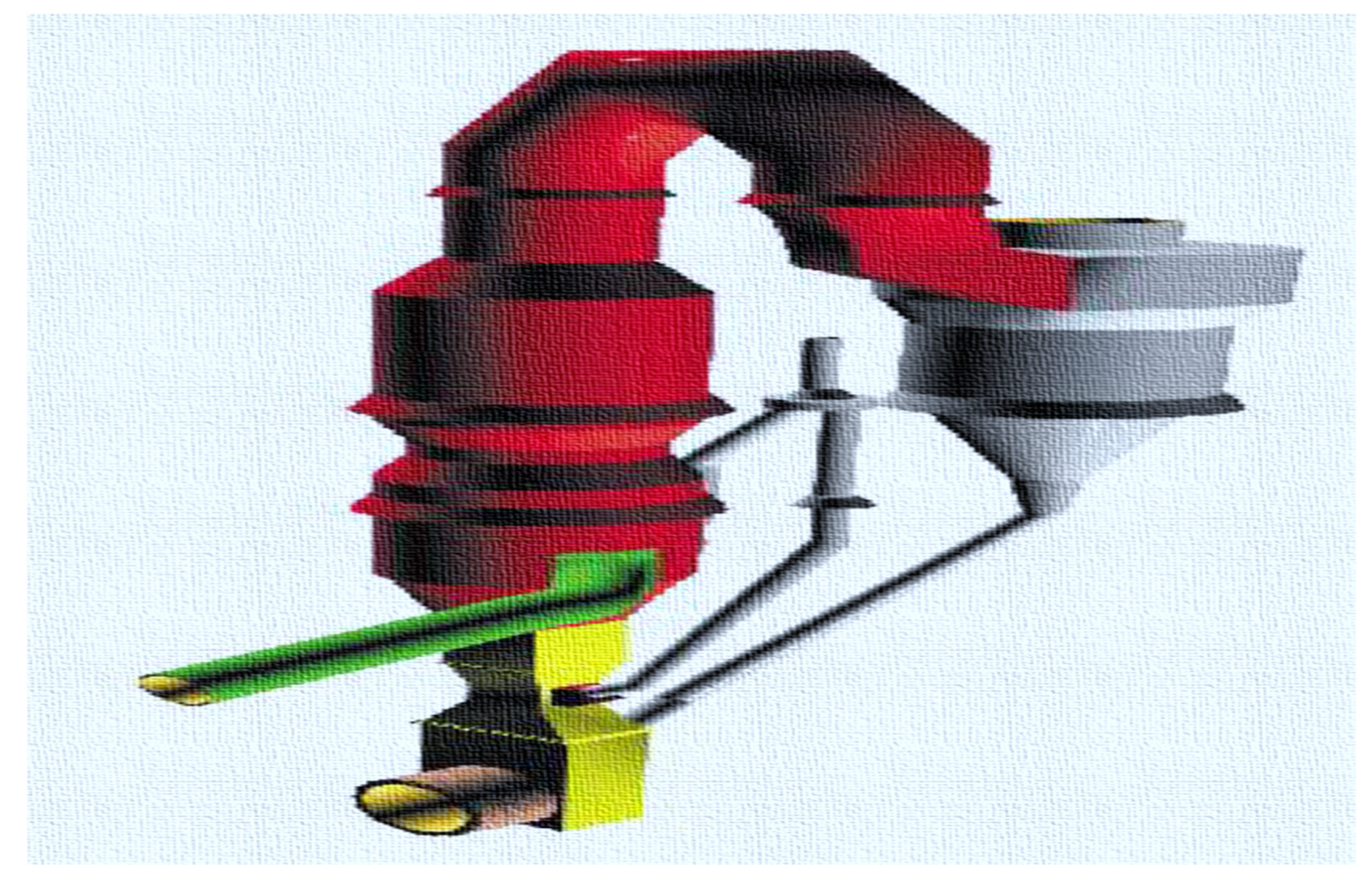The image features a detailed, 3D-like painted diagram set against a textured white fabric canvas background. The foreground machine is displayed against a solid light blue backdrop, adding contrast to its intricate details. To the right, there is a gray, funnel-shaped reservoir that connects to a curved red tube, making a U-shaped bend before feeding into a yellow, angular pump-like system positioned towards the bottom. Attached to this pump is a brown cylinder with a yellow interior on its side. Extending from the top of this yellow section is a green tube pointing to the left, which is connected through at least two round sections. These sections lead to another red tube arching upwards and connecting back to the initial gray funnel. The painting is highly precise, showcasing the mechanical connections with great detail.